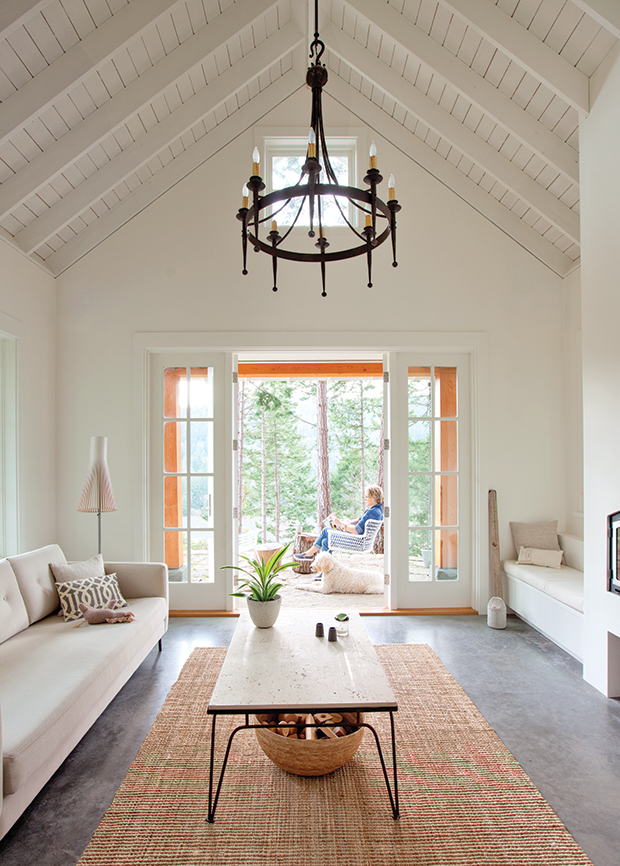The photograph captures the interior of a spacious, two-story room with vaulted ceilings and a peaked roof, all painted in an off-white color. Horizontal and vertical beams are visible on the ceiling. A prominent black chandelier with decorative danglies hangs from the center. At the far end of the room, an open double-sided door, framed with a white trim and an orange border, leads to the outside. Flanking the door are eight small windows, and above the door at the apex of the roof is an additional small window. 

Through the open door, the view extends to a sparsely populated forest of tall trees with green leaves. A middle-aged woman, dressed in a blue shirt, is seated in a white rocking chair facing the left. In front of her, a white poodle-type dog sits on the ground. 

In the foreground, on the left side of the image, stands a white couch accompanied by a white table with black legs, on which sits a pot with a green plant and several smaller items. Beneath the table, a basket with various contents rests on a brown throw rug. The gray-blue floor extends under the rug. On the right side of the image, another white couch is positioned with a white pillow and a smaller brown and white pillow arranged at one end beside a white lamp. The overall scene combines a cozy, lived-in atmosphere with touches of elegance and nature.